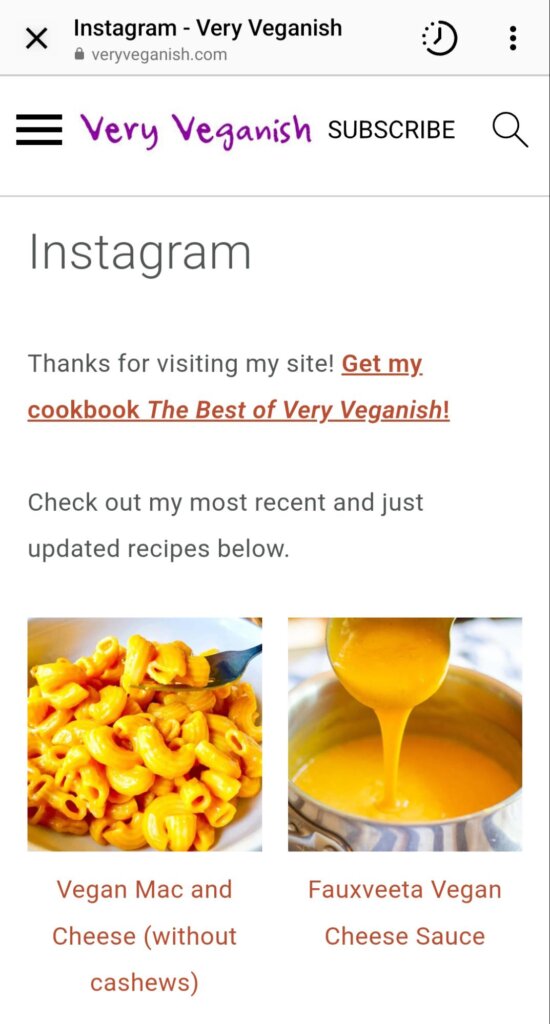This image appears to be a screenshot from a mobile phone displaying a website opened within Instagram. At the top of the screen, there's an Instagram navigation bar showing "Instagram, mine is very vegan-ish," accompanied by a lock icon indicating security, with the URL "veryveganish.com." In the top left corner, there is an "X" icon for closing the window, while the right side features a history icon and a three-vertical-dots menu icon.

Below the navigation bar, the web page content is visible. A menu icon comprising three horizontal lines is positioned at the top, followed by a magenta-colored, handwritten-style text reading "Very Veganish." Directly beneath it, in uppercase gray, sans-serif text, the word "SUBSCRIBE" is displayed next to a search icon. 

A gray horizontal line serves as a divider, under which the word "Instagram" appears in a heading font. The body text below reads: "Thanks for visiting my site." An orange link text invites readers to "Get my cookbook, The Best of Very Veganish." Additional body text encourages visitors to "Check out my most recent and just updated recipes below."

The page features two images of recipes. The left image showcases vegan macaroni and cheese, depicted by a fork holding up some noodles from a white bowl. The caption underneath this image reads "Vegan Mac and Cheese (without cashews)." The right image displays a spoon pouring nacho cheese into a blue and white bowl, captioned "Fovita Vegan Cheese Sauce."